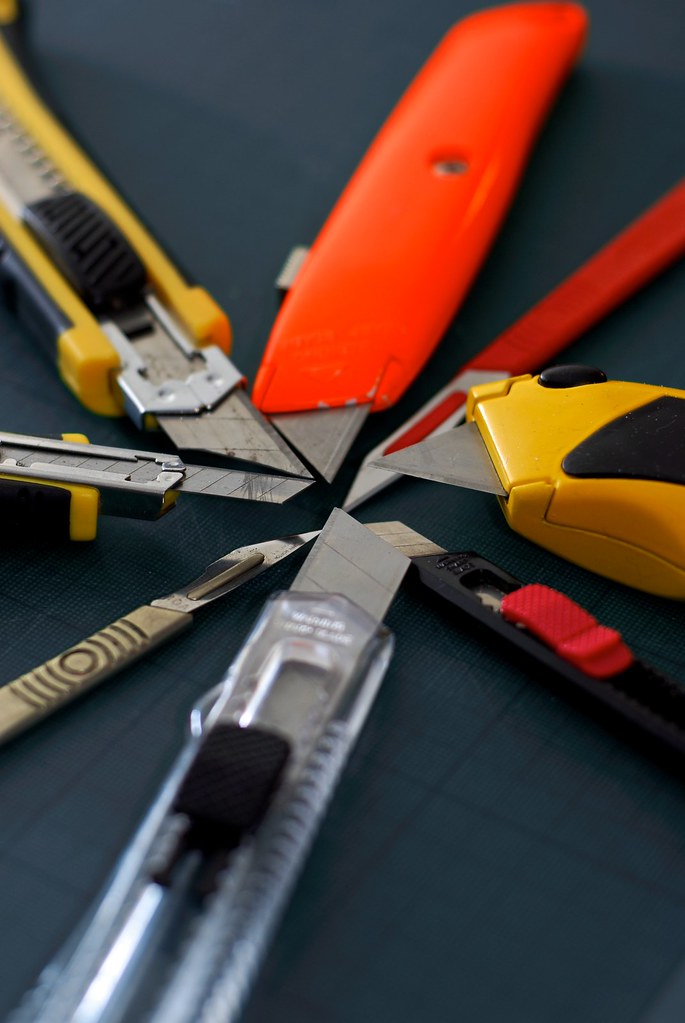This vertically oriented, detailed color photograph captures a striking starburst arrangement of various utility and razor knives, all with their blades prominently extended towards the center. The composition includes an assortment of knives: an orange utility knife, a black and yellow razor knife, a thinner orange razor knife at the top, and a black and yellow utility knife along with a black razor knife featuring an orange knob to the right. At the bottom, a clear acrylic razor knife with a black knob stands out, while on the left side, a knife with a carved wooden handle juxtaposes another with a black and gold handle. All the knives, showing signs of slight wear and screw holes, are meticulously placed on a green gridded cutting surface, creating a visually arresting, almost artistic effect reminiscent of a Chinese star, with their handles radiating outward and partially cropped by the image's edges.